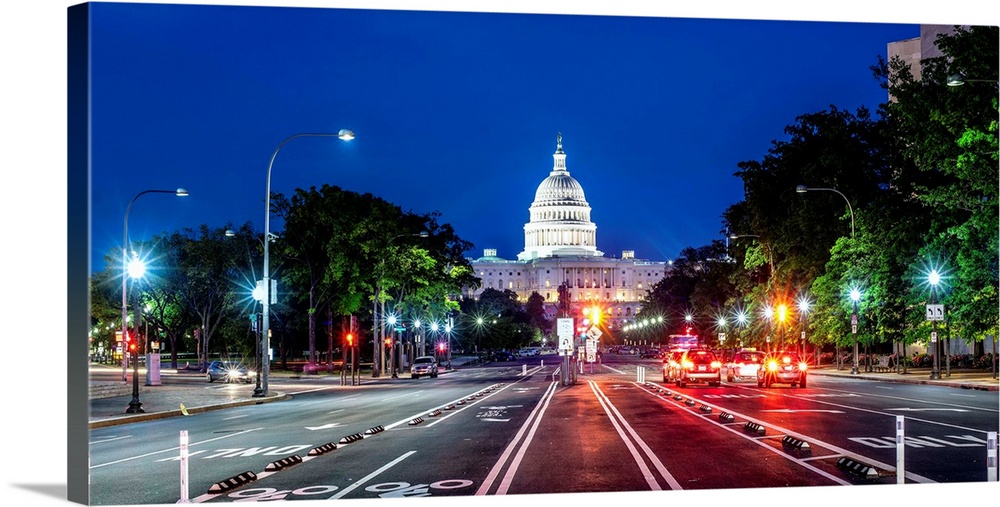In this evocative nighttime photograph of the Capitol Building in Washington, D.C., the scene captures a vibrant and meticulously detailed urban landscape. The dark blue, clear sky forms a dramatic backdrop as the white dome of the Capitol stands prominently, illuminated by bright, white lights. The Capitol building itself is glowing, with various floors lit up, adding depth and grandeur to the structure. 

The photograph appears to have been taken from a vantage point in the middle of a street that leads directly to the Capitol. The street is lined with green trees under streetlights, which add a shimmering neon quality to the scene, possibly enhanced by a recent rain, making the pavement gleam. The streetlights and traffic lights, predominantly green, along with a few cars whose brake lights and headlamps contribute additional points of brightness, emphasize the vibrant play of lights against the night.

On the road, several lanes are visible: on the left-hand side, there's a parked car and lanes designated for bikes and straight traffic; on the right, there are multiple left-turn-only lanes and a straight-ahead lane. Beyond the trees lining the street, a few buildings peek over, with one notably visible on the right-hand side. The composition, possibly akin to a stretched poster, accentuates the light and reflections, creating a scene rich in shimmer and urban energy, ultimately highlighting the Capitol in a striking, almost cinematic distance.